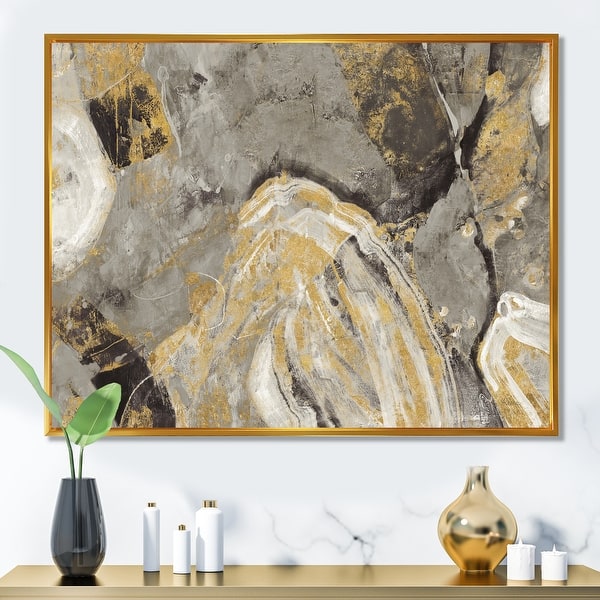The image presents a meticulously arranged scene within a square frame, focusing on a section of an interior wall that appears to be crafted from predominantly white marble with subtle grey veining. At the bottom of the image, a gold, reflective shelf spans the width of the frame, partially cropped by the image's edges. 

The central feature of this arrangement is a rectangular painting housed within a frame that boasts a gold band. The painting itself is abstract, displaying a textured pattern that echoes natural rock formations with a palette that includes browns, dark greys, lighter greys, and hints of near-black, suggesting the appearance of mountain peaks and vast cracks.

To the left of this framed artwork, a black conical vase holds two green leaves, their stalks partly obscuring the painting. Adjacent to this on the shelf are three cylindrical white decorations, adorned with thin gold accents. To the right, a gold conical vase with a wide middle and narrow neck stands empty but reflective. Further to the right, two round white candles of different heights, each with visible wicks, complete the arrangement.

Together, these elements form a sophisticated and harmonious display, blending natural textures with reflective gold accents and minimalistic decorations, all anchored by the striking abstract painting central to the composition.